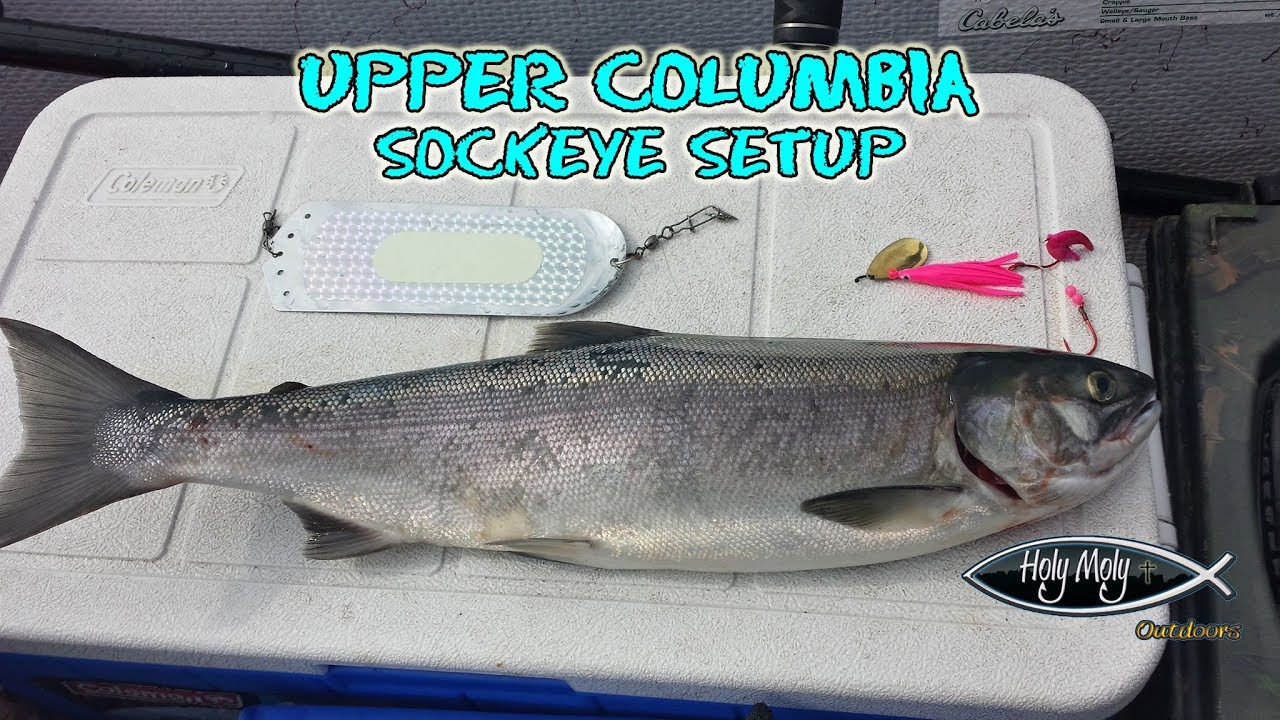The image features a recently caught whole salmon with a silver-greenish hue, lying on top of a standard white-topped, blue Coleman cooler. Centered on the cooler's lid is a light blue text with a gray border that reads "Upper Columbia Sockeye Setup," along with a white tag positioned near the text. To the right of the tag, a bright pink fishing lure and another piece in yellow are visible. Near the fish's head, there's a fish-shaped logo with a black interior and a silver border that reads "Holy Moly" in white, followed by partially obscured text. The background appears to consist of a padded gray surface, likely the interior of a boat. Notably, the lower right corner near the logo includes a stamp that indicates the brand "Holy Moly Outdoors," identified by a fish symbol with a cross. A black fishing rod is also faintly discernible in the background, and small decorative elements such as flowers could be on or around the cooler. There are no people visible in the photo.